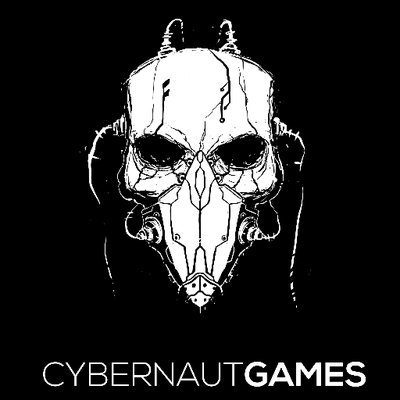The image is a striking black and white square, featuring a central drawing of a skull adorned with a futuristic, cyberpunk-inspired mask. The skull, predominantly white with black detailing, has empty, slightly cracked eye sockets and a nose component that appears to be clipped or screwed onto its structure. Black lines reminiscent of computer motherboard circuits run across the skull, enhancing its high-tech appearance. White wires emerge from the top and sides of the mask, suggesting a connected, mechanized system. The mask itself replaces the lower jaw of the skull and lacks air holes, adding to its eerie and mechanical aesthetic. Below the skull, in bold, capitalized sans-serif text, is the inscription "CYBERNAUT GAMES," which stands out starkly against the pure black background. This haunting and intricate design likely serves as the company’s logo, embodying a blend of horror and advanced technology.